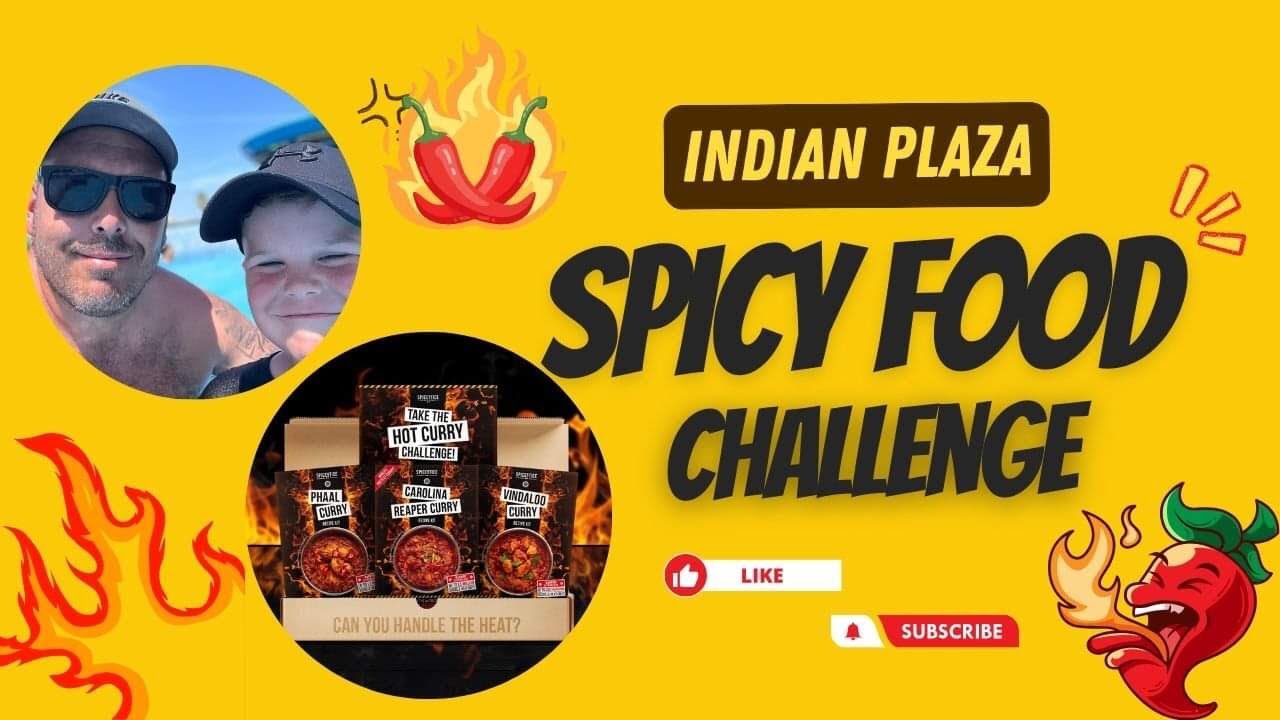The image features a rich goldish-yellow background with fiery elements, emphasizing the theme of heat and spice. At the top, two red peppers are engulfed in flames, creating a dramatic centerpiece. The upper right corner proudly displays a brown rectangle with rounded corners, within which "India Plaza" is written in vibrant yellow letters, and "Spicy Food Challenge" is inscribed below in bold black text.

On the bottom left, there's a complex outline of a red flame, adding to the fiery theme. Opposite, in the bottom right, an animated red pepper character is blowing out smoke, signifying intense heat; it has expressive closed eyes and a mouth, facing left.

Two circles containing images are placed on the upper left. In the first circle, a man and a boy, both wearing hats with water and blue sky in the background, are visible. The second circle depicts three bags of food items, likely hot curry-flavored snacks. Accompanying text near these images reads, “Can you handle the heat?” and “Take the hot curry challenge.”

Situated at the bottom right corner are interactive elements: a red circle with a white thumbs-up icon inside, accompanied by a white rectangle tagged "Like" in red. Additionally, there's a stylized white square, pointed at one end with a bell icon inside, and a uniquely shaped rectangle with white text that reads "Subscribe."